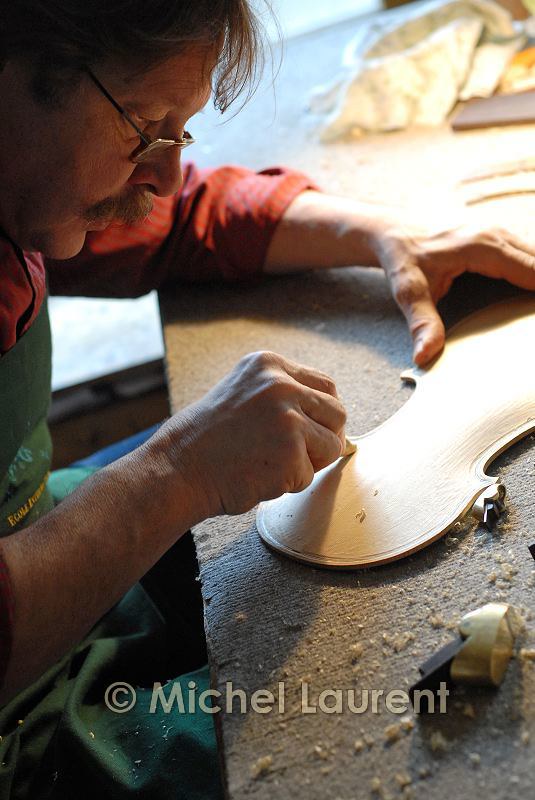The photograph depicts an older Caucasian luthier deeply engrossed in carving a piece of light-colored wood, which likely belongs to a stringed instrument such as a violin or guitar. Situated at his work desk covered in wood shavings and tools, he wears glasses, a red long-sleeved shirt, and a green apron adorned with some printing. With concentrated effort, he holds the wooden object with his left hand while carving with his right, revealing a pattern resembling a violin's wing or a guitar head. The work desk, with a tan cloth on top and bits of crumbled wood, supports various light-brown wooden parts around the edges. The image is credited to Michel Laurent, potentially the photographer or the subject of the photograph.